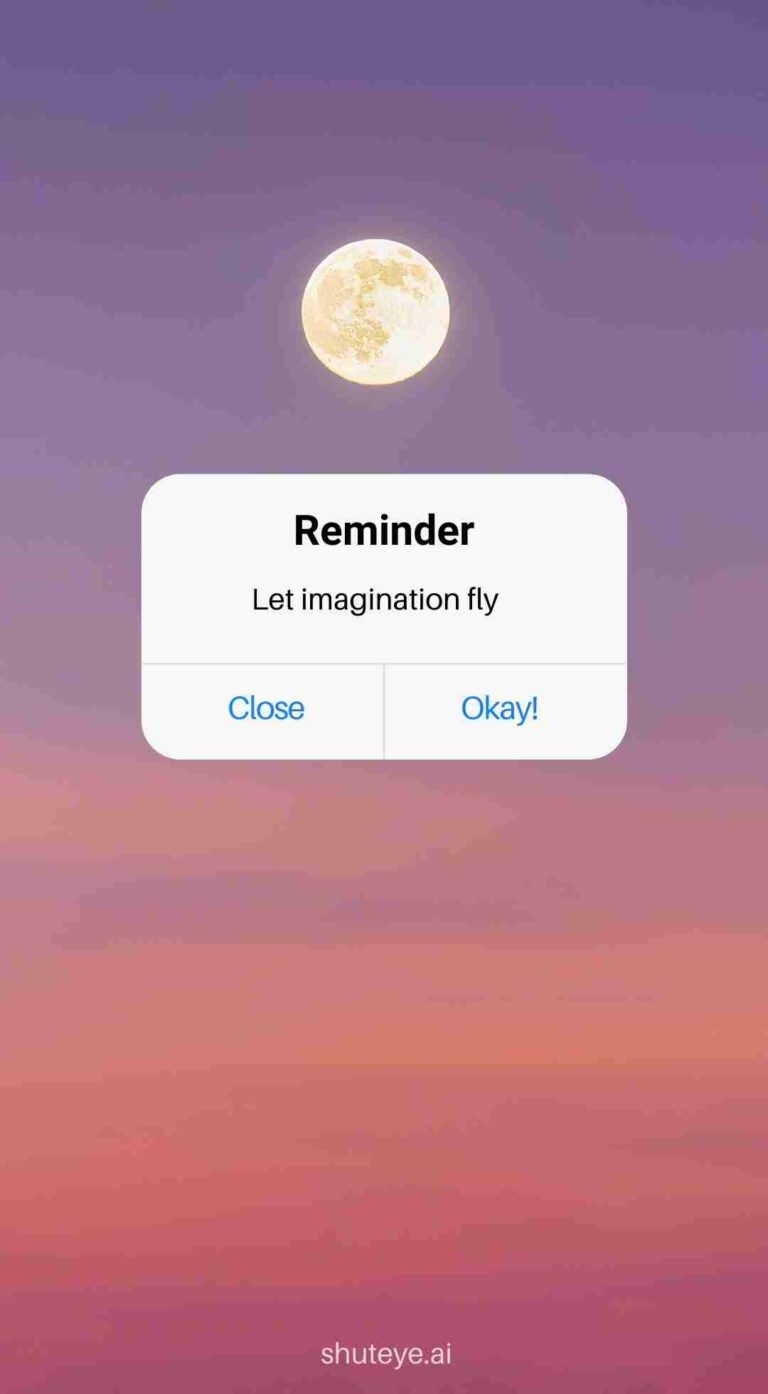This image is a screenshot taken from a cell phone, featuring a stunning abstract artwork as the background. The top portion of the image captures the vibrant colors of a sunset sky, depicted through a series of wavy horizontal lines. These lines transition from a deep plum purple at the top, gradually lightening to a beautiful lavender hue. As the colors continue downward, they blend into an exquisite swirl of orange and pink shades. A large, bold strip of orange dominates the middle section, followed by deep orange hues interspersed with pinks, reds, and dark purplish-pinks towards the bottom of the screen. Central to the image is a bright, round white moon with a yellow glow above it. Superimposed over the abstract background, a white rectangular notification box features the word "Reminder" in bold black text, with the phrase "Let Imagination Fly" in blue text beneath it. At the bottom of the notification box are two options: "Close" and "OK."